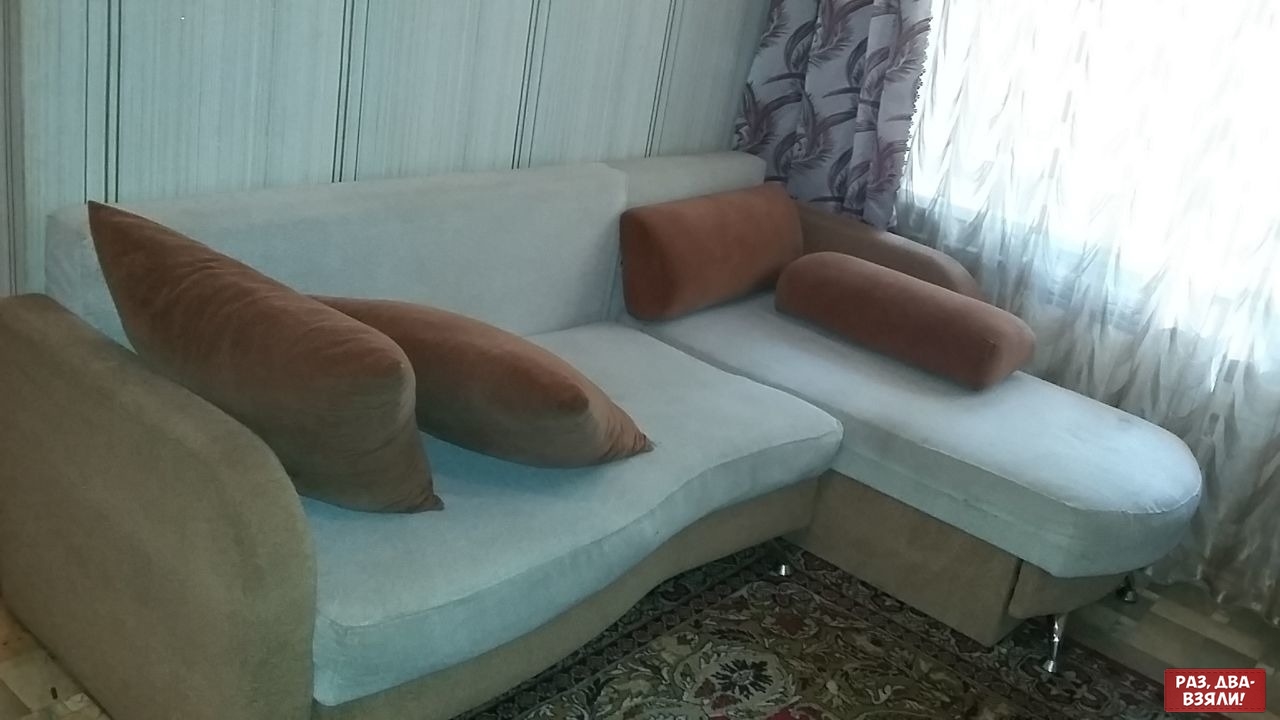This detailed image captures a living room scene centered around a prominent L-shaped couch, which appears to dominate most of the photograph. The couch is primarily white with a grayish felt covering the bottom section and features an extended footrest on one side. It is accessorized with a mix of brown-ish gold and red throw pillows, some descriptions also suggesting blue cushions. The backdrop includes a rectangular window adorned with light blue drapes combined with darker blue and white accents, accompanied by a sheer white curtain that allows sunlight to stream in. The floor showcases a richly patterned throw rug with a complex design featuring red, gold, and black hues. Behind the couch, the wall is either light blue or unremarkable, and the natural lighting, despite being sunny, gives a balanced illumination to the slightly darker interior.